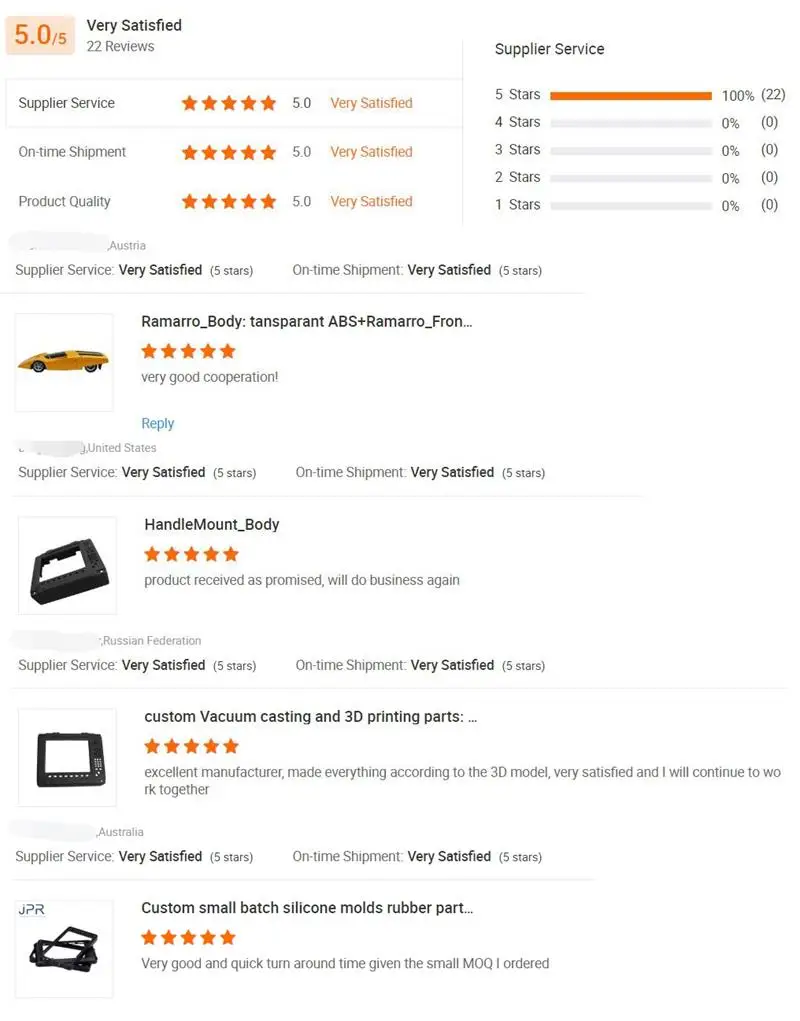This screenshot captures a review page boasting an impeccable 5.0/5 rating, indicating high customer satisfaction across 22 reviews. At the forefront, the page showcases consistent top ratings for key performance aspects: Supplier Service, On-time Shipment, and Product Quality, each adorned with dark orange five-star icons and labeled "5.0" and "Very Satisfied" in a lighter orange hue.

To the right of this evaluation box, a detailed breakdown of Supplier Service demonstrates that 100% of the 22 reviewers awarded five stars, highlighted by an elongated orange bar beside the highest rating.

Below this summary, the page features images and corresponding reviews of various products available on the website:
1. An orange model car described as "Romaro body transparent ABS plus Romaro_front," rated five stars with a note of "Very good cooperation."
2. A black box identified as "Handle mount_body," also rated five stars, with a comment stating "Product received as promised. We'll do business again."
3. Another black item named "Custom vacuum casting and 3D printing parts," though lacking an individual review comment.
4. A final product listed as "Custom small batch silicone molds rubber," similarly featured without specific reviewer feedback.

The screenshot succinctly conveys a strong sense of reliability, quality, and customer satisfaction through its visual and textual elements.